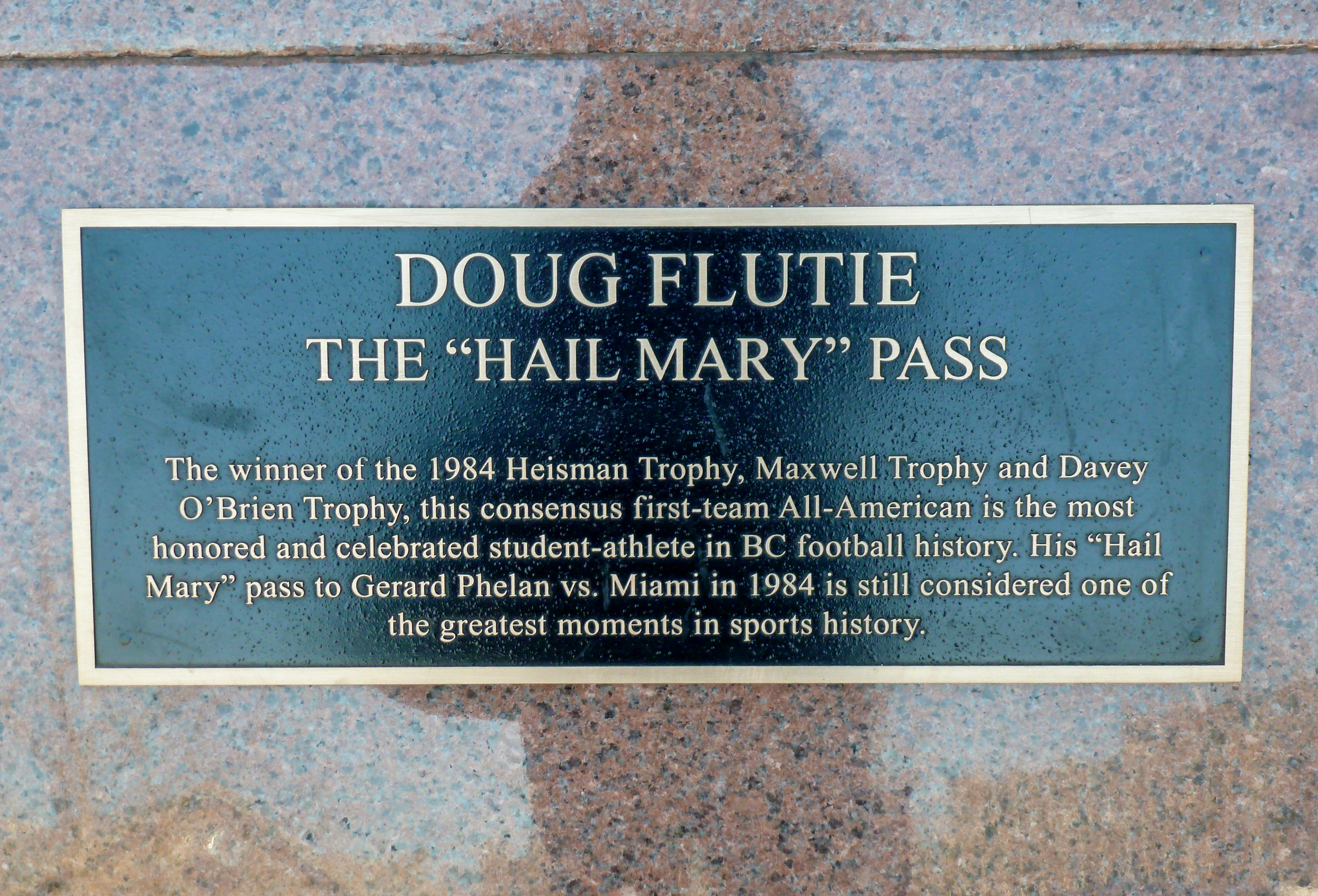The image depicts a color photograph of a metal plaque that is mounted on a highly polished, speckled granite wall, characterized by pink, black, and white hues. The plaque itself features a black background with gold uppercase lettering and is bordered in a gold trim. The top of the plaque prominently displays "Doug Flutie, the Hail Mary Pass" in large gold letters. Below this, in smaller text, it reads: "The winner of the 1984 Heisman Trophy, Maxwell Trophy, and Davey O'Brien Trophy. This consensus first team All-American is the most honored and celebrated student-athlete in BC football history. His Hail Mary Pass to Gerard Phelan versus Miami in 1984 is still considered one of the greatest moments in sports history." The photograph is well-lit, showcasing the clear details and contrast of the plaque, with the shadow of the photographer faintly visible on the reflective granite surface.